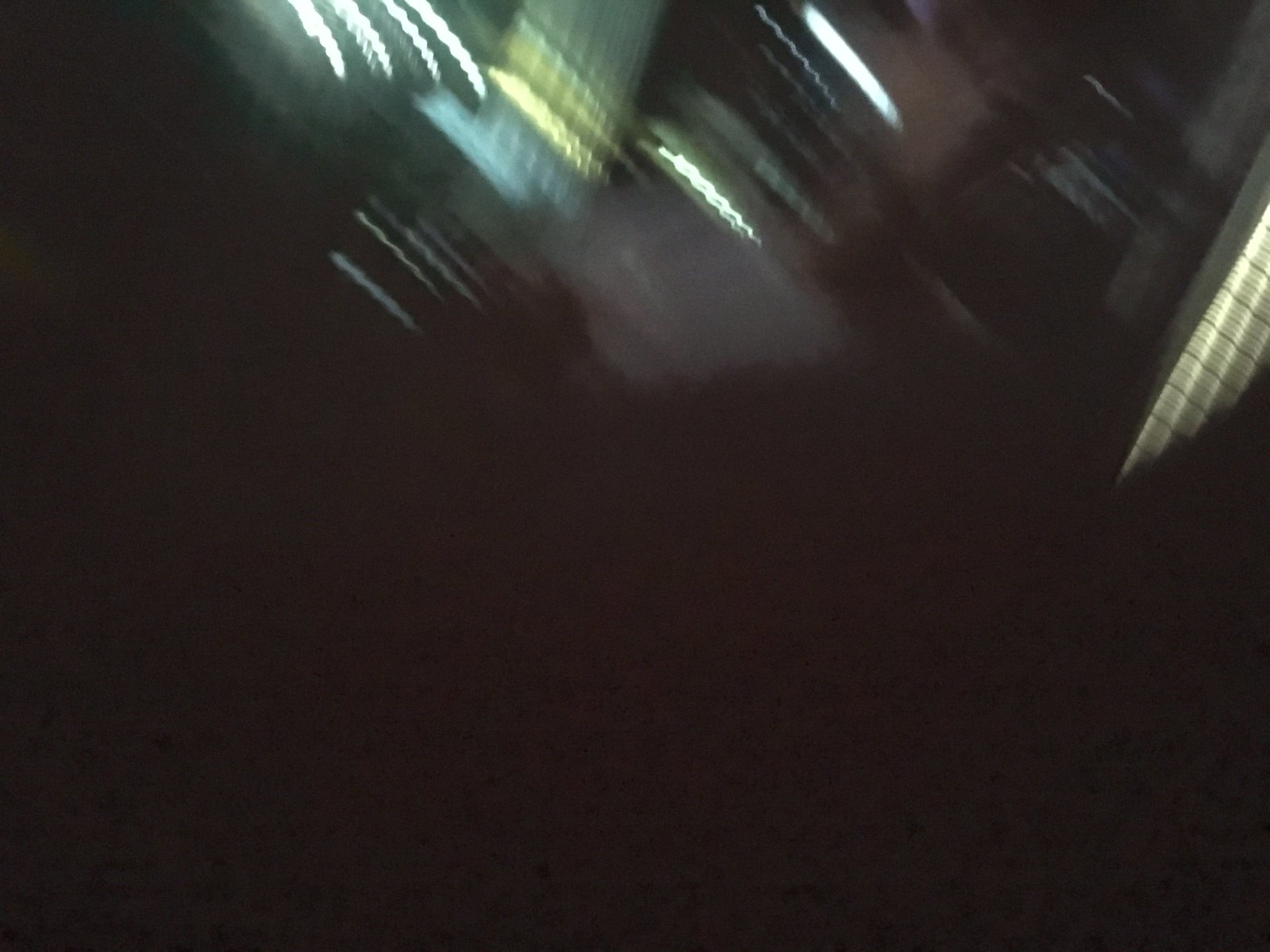The image appears to be a night-time photograph that is heavily blurred and out of focus, giving it an abstract art-like quality. The top of the image features various blurred objects that may be metallic or illuminated, creating distorted light patterns. These objects include a mix of colors such as dark brown gradating to black, blue-green with white ripply lines, lighter green, yellow, and light blue streaks. Additional features include light blue rectangles, dark green, and light gray squiggly lines. On the right side, there are patches of green transitioning to lighter green with white squiggly lines, under a gray patch and a white bar. The bottom half of the image is predominantly dark brown with gray lines and patches, interspersed with greenish-gray and yellow with green stripes. Overall, the image is characterized by its highly blurred lights and indistinct shapes, resembling smudged lights perhaps captured while the camera was being moved.